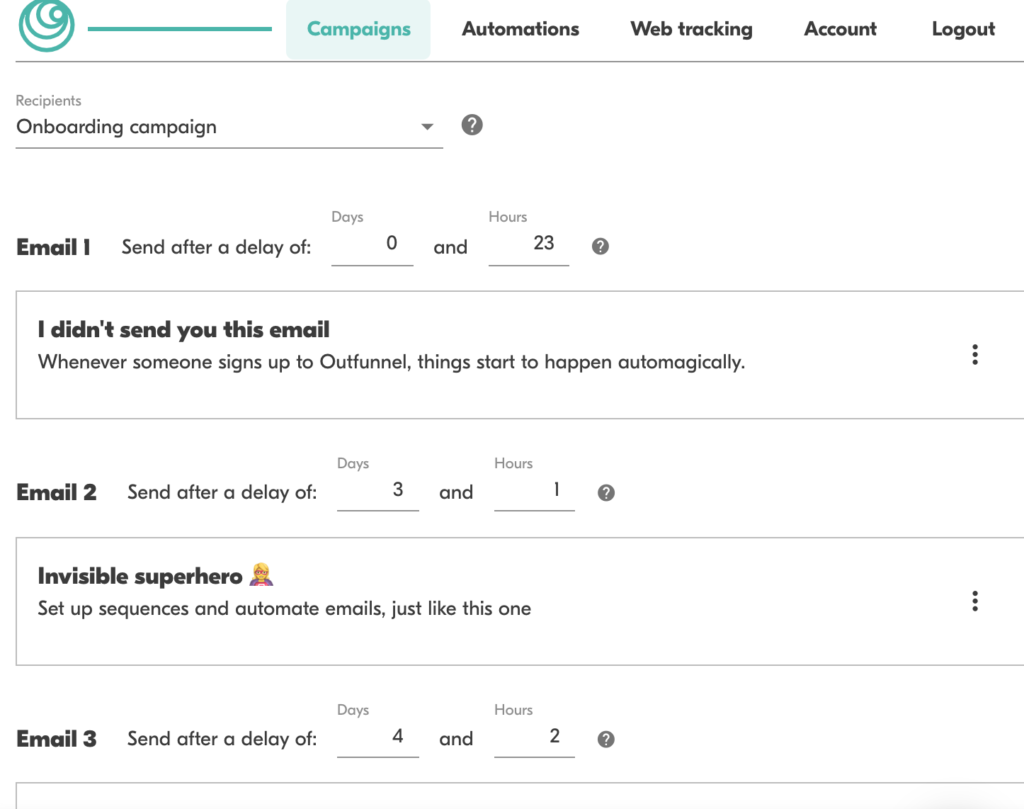This is a detailed and cleaned-up caption for the described image:

---

The screenshot features the interface of a website, displaying various navigation categories at the top right corner, including "Campaigns," "Automations," "Web Tracking," "Account," and "Logout." Below this section, on the left side, the screen lists "Recipients" and "Onboarding Campaign."

Within the "Onboarding Campaign," the progression of automated emails is detailed as follows:

- **Email 1**: Sent after a delay of 0 days and 23 hours. This email contains a box with the text: "I didn't send you this email, whenever someone signs up to Outfunnel, things start to happen automagically."
- **Email 2**: Sent after a delay of 3 days and 1 hour. It includes a message about being a "visible superhero," with instructions on setting up sequences and automating emails like the one being viewed.
- **Email 3**: The header of this email is partially visible, showing that it is sent after a delay of 4 days and 2 hours, accompanied by a small circle with a question mark inside it.

---

This cleaned-up caption provides a clear and detailed description of the screenshot contents, conveying the structure and purpose of the displayed elements.